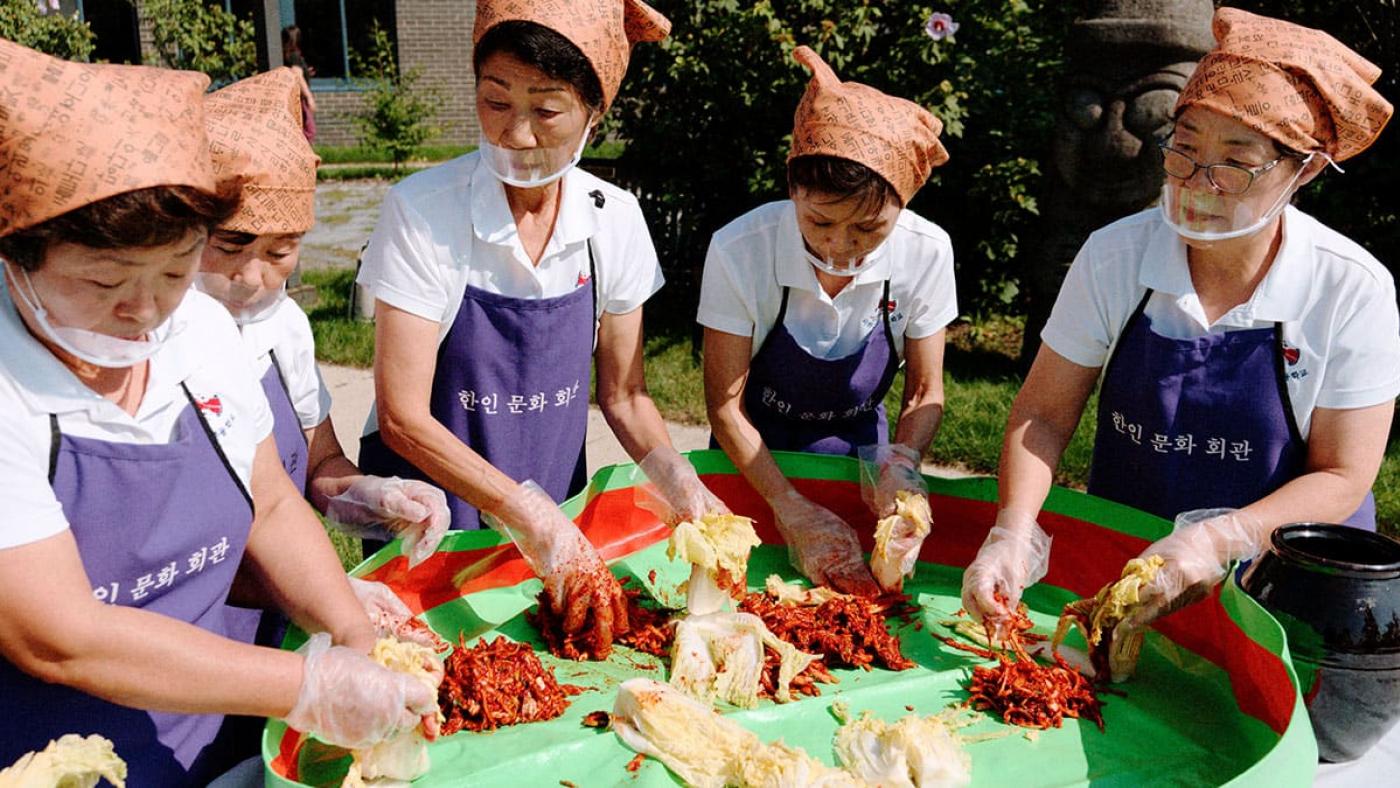The photograph captures five women, likely of Asian descent, standing in a semicircle around a small kiddie pool atop a table. They are identically dressed in white shirts adorned with a red logo on the left breast, lilac-colored aprons featuring Asian characters across the center, and peach-colored scarves covering their hair. Each woman also dons a surgical-style face mask with a clear opening, along with clear plastic food safety gloves on their hands. The women are seen manipulating a red mush formed into balls, which appears to be kimchi preparation. Some wonton wrappers are also visible in the center of this green circular vat. In the background, bushes including a rose of Sharon can be seen, adding to the outdoor setting.